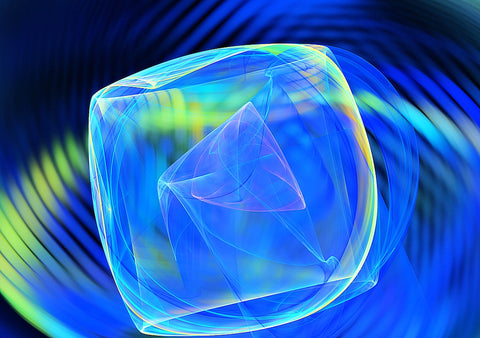The image is a digital illustration characterized by its abstract and surreal nature. At the forefront, it features a semi-transparent, rounded cube or a rounded square shape, resembling a cube with tesseract-like qualities that internal polyhedron seemingly moves within. This central shape is primarily blue with hints of purple and light green, giving it an opalescent appearance reminiscent of a gemstone. Swirling and curving through and around it are white-yellow lines that resemble diffuse light patterns, as if light is being diffracted similarly to how it would through a bubble. In the background, colorful bars swirl in circular wave patterns, predominantly blue but interspersed with yellow, contributing to the image's dreamlike quality. The entire image utilizes computer-generated graphics to create a mesmerizing and dynamic play of colors and shapes that evoke a folded reality.